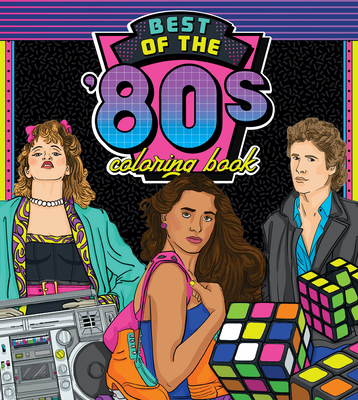The cover image for the "Best of the 80s Coloring Book" is a detailed and vibrant homage to the iconic era. Against a black background, a distinctive blue border with pink, purple, yellow, and blue stripes frames the cover. Prominently at the top, the title "Best of the 80s Coloring Book" is displayed. 

On the far left stands a woman with shoulder-length, light brown hair, adorned with a pink bow, wearing a blue jacket over a black top, reminiscent of Madonna. She poses with a confident, no-nonsense demeanor. The bottom left corner of the cover features a silver boom box, capturing the essence of 80s music culture.

At the center of the image, another woman draws the viewer's attention directly to the camera. She has long brown hair and carries orange roller skates with teal laces slung over her shoulder, indicative of youthful vibrancy. Her serious and determined expression evokes a sense of purpose and urgency.

On the far right, a man with short, light brown hair wears a blue collared button-down shirt beneath a black jacket, possibly representing Lorenzo Lamas from "Falcon Crest." Completing the vintage aesthetic, the bottom right corner showcases three Rubik's Cubes in lime green, pink, orange, white, yellow, and indigo, with one cube partially cropped, signifying the popular 80s puzzle game.

Altogether, the cover encapsulates the spirit of the 80s with its rich details and nostalgic elements, including resonant 80s celebrities, music, and games.